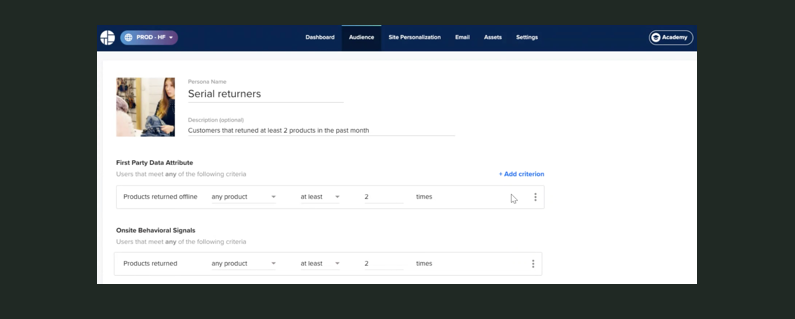The image is a rectangular screenshot with a black background. At the top, there is a dark blue header featuring several menu options in a small white font. These options include "Dashboard," "Audience," "Site Personalization," "Email Assets," and "Settings." Towards the right of the header, there is an oval shape with a white border labeled "Accessibility." Adjacent to this oval, on the left, you can see a circular white icon with an indiscernible blue element in the center, likely due to its small size.

The "Audience" menu option is selected, indicated by a black background, a rectangular shape, and a green line at the top edge of the tab. Below the header, the main section has a white background. In the upper-left corner of this section, there is an image of a woman with golden blonde hair, facing the camera with her left cheek. She is wearing a black shirt and appears to be holding a piece of fabric, possibly a denim jacket. Another individual with gray hair is partially visible to the left of her.

To the right of the image, the text "Personal Name" appears, followed by a prominent black heading that reads "Serial Returners." Beneath this heading, in small gray letters, there is a line labeled "Description (optional)." Following this, in slightly larger but still smaller black text compared to the header, it states, "Customers that returned at least 2 products in the past month," where the number "2" is written as a numeral.

Further down on the left side, there is a line of small black bold text that reads "First Party Data Attribute." Below this, in small gray lettering, it explains, "Users that meet any of the following criteria," with the word "any" emphasized in bold.